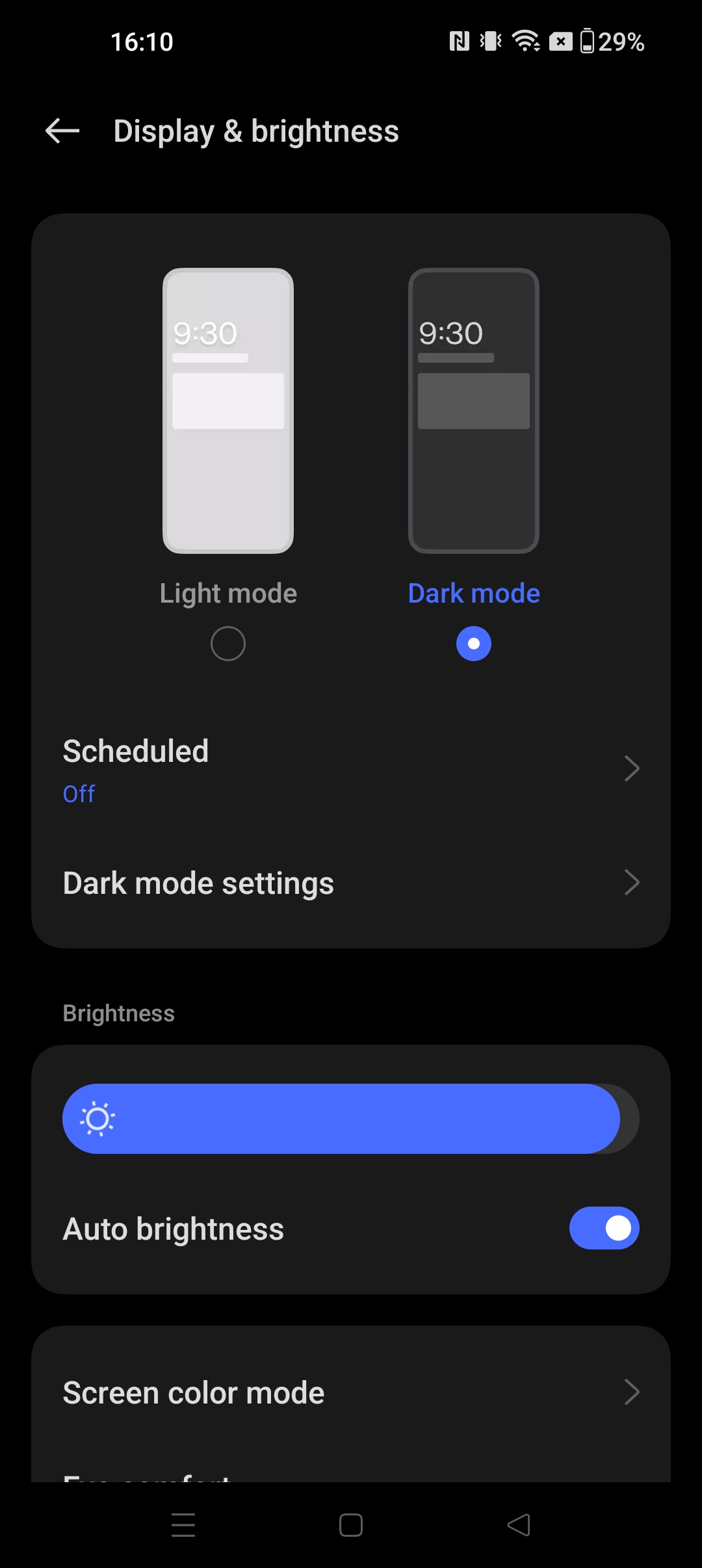This image is a detailed screenshot of a smartphone's "Display and Brightness" settings. The screen background is black, with most of the text in white for readability. 

At the very top of the screen:
- The time is displayed on the top left as "16:10."
- The top right corner contains various system icons: the phone is on vibrate mode with the sound muted, Wi-Fi connectivity is active, and the battery level is at 29%. 

Below the status bar:
- A left-pointing arrow indicates a back navigation option.
- The heading "Display and Brightness" is prominently displayed.

Following this, the display mode choices are shown:
- Two icons representing phones, one in white (light mode) and another in dark gray (dark mode), are displayed.
- "Dark Mode" is selected, highlighted in blue to indicate the active choice.

Under these options:
- The "Scheduled" setting is shown as toggled off.
- An option labeled "Dark Mode Settings" is available.

Next comes the brightness adjustment options:
- The "Brightness" section shows that auto-brightness is enabled.
- The brightness level slider is nearly full.

Further down:
- The "Screen Color Mode" option is available with a right-pointing arrow indicating additional settings.

Finally:
- The bottom of the screen shows three navigation icons: three horizontal bars, a white square, and a white left-pointing triangle inside a black bar.

This comprehensive view of the device's display settings confirms the selection of dark mode with high brightness and full Wi-Fi connectivity.